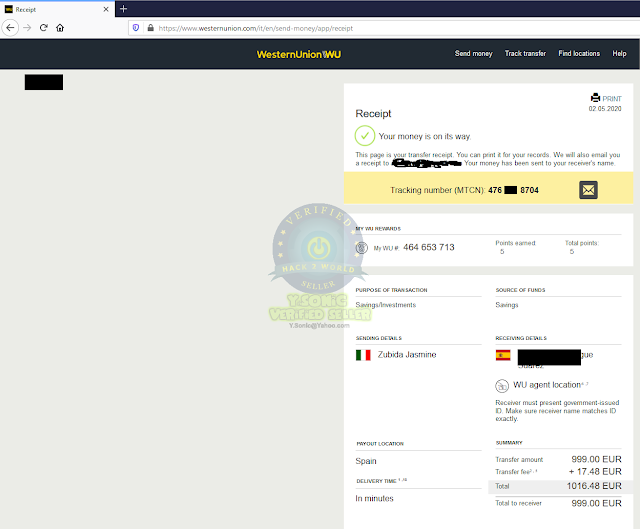The image displays a tab on a live web page from WesternUnion.com, specifically the "Send Money" section. The page showcases a confirmation receipt for a completed transaction. Key elements of the page include an option to print the receipt and a watermark indicating verification as a "HAC 7 World Seller."

The receipt conveys the message: "Your money is on the way. This page is your transfer receipt. You can print it for your records. We also email you a receipt." The email address associated with the receipt is obscured. The receipt confirms that the money has been sent to the receiver, whose name is not visible.

A tracking number is provided: MTCN 7476 **** 8704. The transfer amount is specified as 999 Euros, and the destination is Spain. The source of the funds is marked as "Savings," with the purpose noted as "Savings and Investments." The sender's details list the name Zubida Jasmine, while the receiver's details are censored. 

Overall, the image captures a detailed, active confirmation page for a money transfer on the Western Union website.